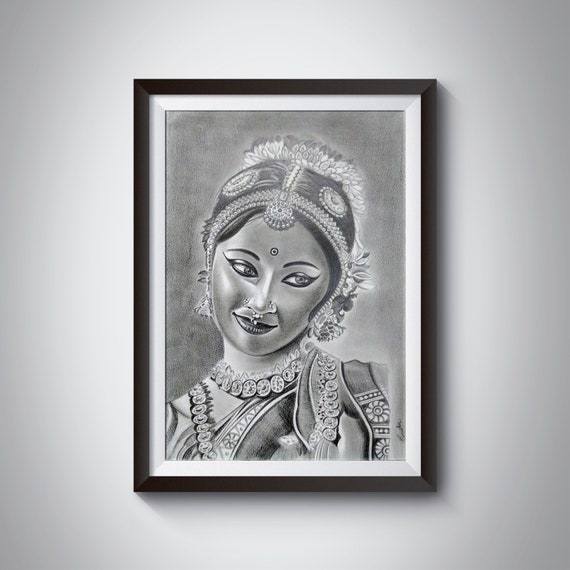This image features a detailed black-and-white pencil sketch of an Indian woman, framed and hanging on a gray and white wall. The frame is black with a white inner border. The woman in the drawing is depicted from the chest up and is adorned with intricate traditional attire. Her elaborate headpiece covers most of her hair, embellished with ornaments and flowers, leaving a few strands peeking out in the front. She wears a distinctive bindi on her forehead, along with extensive eyeliner that extends to the outer corners of her eyes and sharply defined eyebrows. Her nose is adorned with both a nose ring and a hoop piercing, and she flaunts bold, dark lipstick. She is dressed in a traditional blouse and an intricate neckpiece featuring circular embellishments that extends down past her neck. The woman, with an air of grace, gazes toward the bottom left corner of the picture, smiling subtly with her mouth closed, capturing a timeless beauty accentuated by her ornate jewelry and makeup.